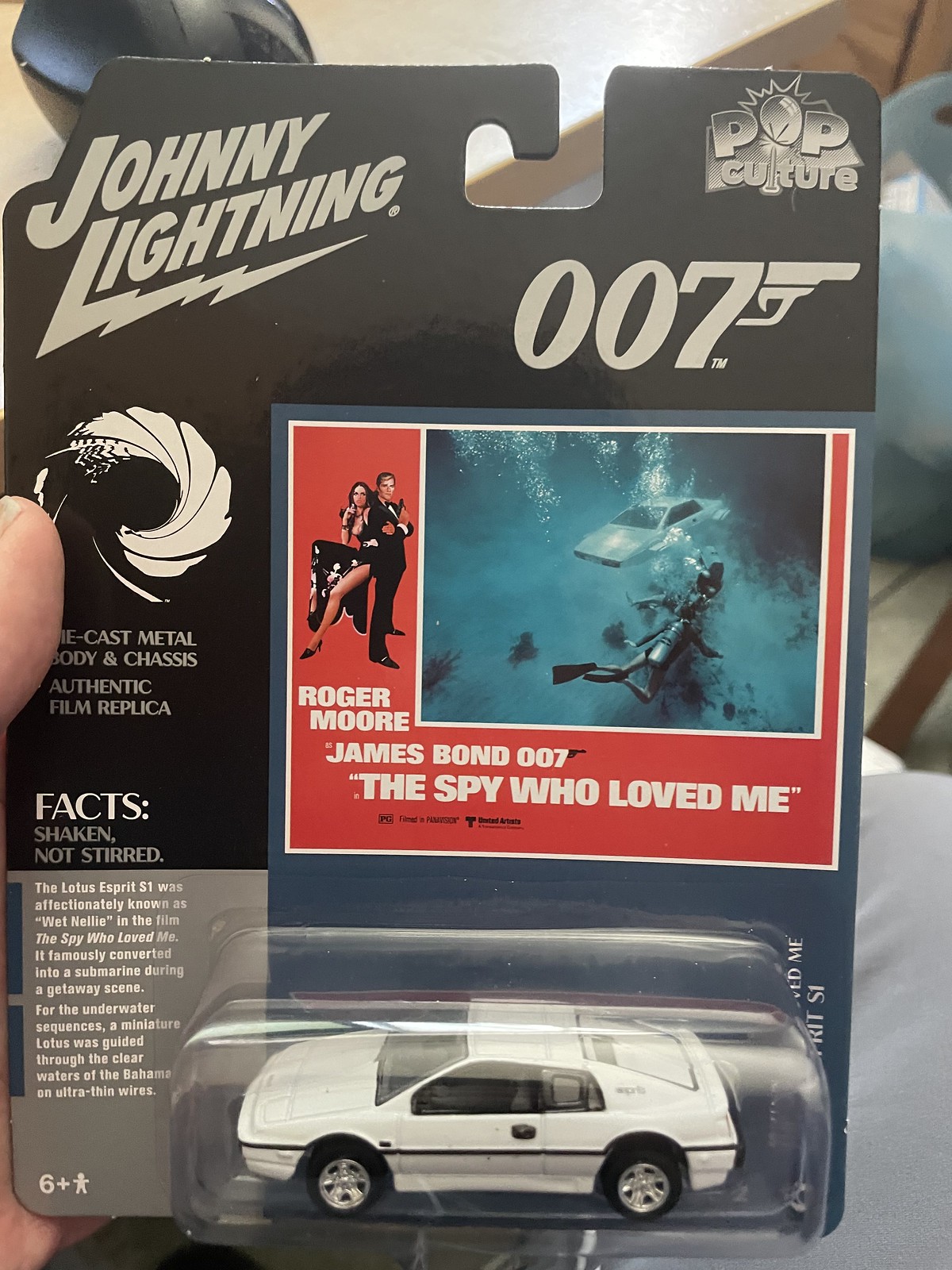This vertical rectangular image features a package for a mini toy car, replicating the white sports car used in the James Bond movie "The Spy Who Loved Me." The package, held by a person whose fingers are visible, has a top-notch for hanging on a rack and sports a gray background with an indistinct object visible behind it, possibly office furniture.

At the top left of the package, the brand "Johnny Lightning" is prominently displayed, with the L in "Lightning" creatively extending into a lightning bolt. The top right showcases the "Pop Culture" logo, and just below it, the iconic "007" trademark, incorporating the handle of a gun into the numerals.

In the center of the package, a red rectangle features an illustrative scene from the film, depicting Roger Moore as James Bond, accompanied by a woman, against an underwater backdrop with scuba divers and the car in its submarine mode. Underneath this scene, the text reads "Roger Moore, James Bond 007, The Spy Who Loved Me."

Encased in plastic at the bottom of the package is the detailed toy car, labeled as having a cast metal body and chassis, boasting authenticity as a film replica. The package also highlights the famous Bond quote "Shaken, not stirred," adding to the nostalgic appeal for collectors and fans of the franchise.